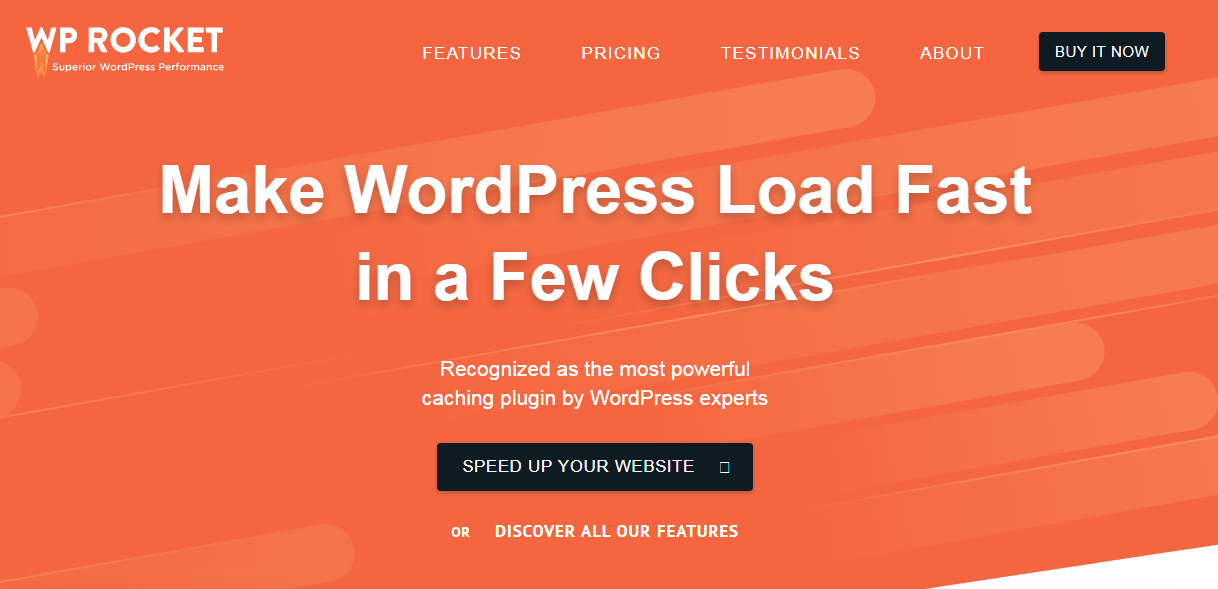The image features a predominantly reddish-orange background with white text and design elements. In the top left corner, the white text reads, "WP Rocket," accompanied by the tagline, "Superior WordPress Performance." On the top right, there are navigation tabs labeled "Features," "Pricing," "Testimonials," and "About," all in capital letters and white text.

A prominent black button on the top right corner bears the inscription "BUY IT NOW" in white text. Centrally positioned, bold white text declares, "Make WordPress Load Fast in a Few Clicks." Below this, smaller white text states, "Recognized as the Most Powerful Caching Plugin by WordPress Experts."

Further down, another black button with white capital text reads, "SPEED UP YOUR WEBSITE," positioned next to a small white box. Under this, the text "OR" appears in capitals, followed by "Discover All Our Features," all in white text. 

The background features an array of rounded, oval-like shapes ascending towards the upper right of the page. A small, completely white cutoff piece is visible at the bottom right corner of the page, adding a contrasting design element to the layout.